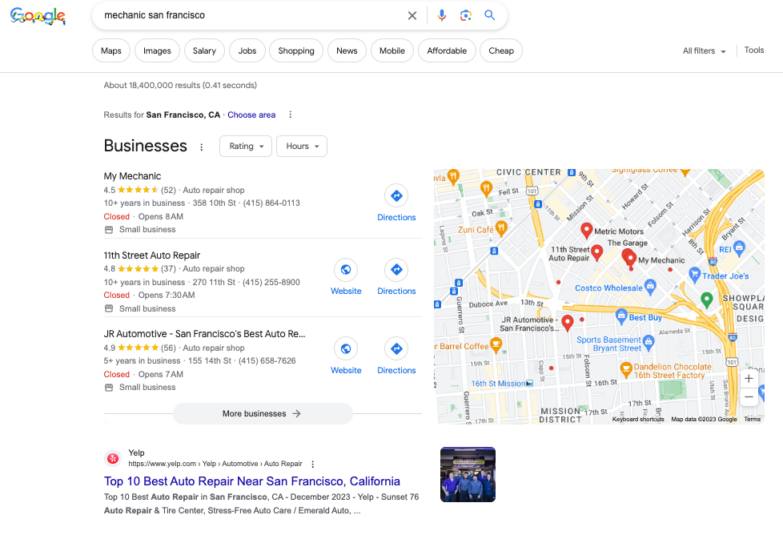A screenshot of a Google search results page is displayed, featuring the Google logo adorned with festive Christmas lights in the top left corner. The search query entered is "mechanic, San Francisco." Directly below the search bar, multiple navigational buttons are visible, including "Maps," "Images," "Salary," "Jobs," "Shopping," "News," "Mobile," "Affordable," and "Cheap."

Beneath these buttons, the page reveals the number of search results found for San Francisco, California, along with the time it took to generate these results. Following this, there is a section listing local businesses, with three specific mechanics highlighted: My Mechanic, 11th Street Auto Repair, and JR Automotive, San Francisco's Best Auto Repair. Each listing notes that the businesses are currently closed and offers clickable links to their websites and directions.

Adjacent to these listings, a small map shows the geographical locations of each mechanic with pins marking their places. At the bottom of the section, a "More businesses" button with a right-pointing arrow suggests that additional mechanic options are available for viewing.